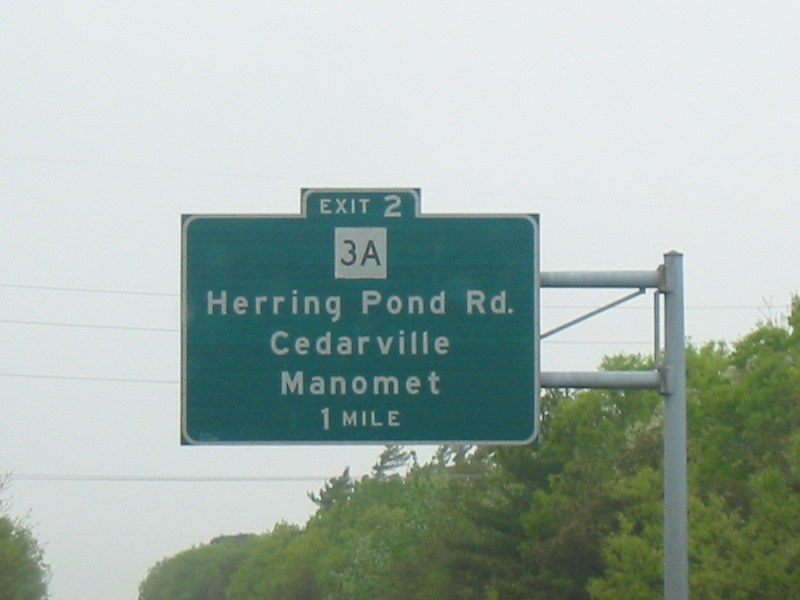This daytime photograph captures a green rectangular highway sign supported by a thick silver pole with two horizontal arms and an angle brace, indicating its substantial size. The sign prominently features white lettering. At the top, a small rectangular section reads "Exit 2" with a small, white square below showing "3A." The main portion of the sign informs drivers of "Herring Pond Road, Cedarville, Manomet" and notes these destinations are "1 mile" away. The scene is framed by treetops with lush green leaves and several horizontal power lines, set against a light gray, overcast sky, suggesting possible impending inclement weather.